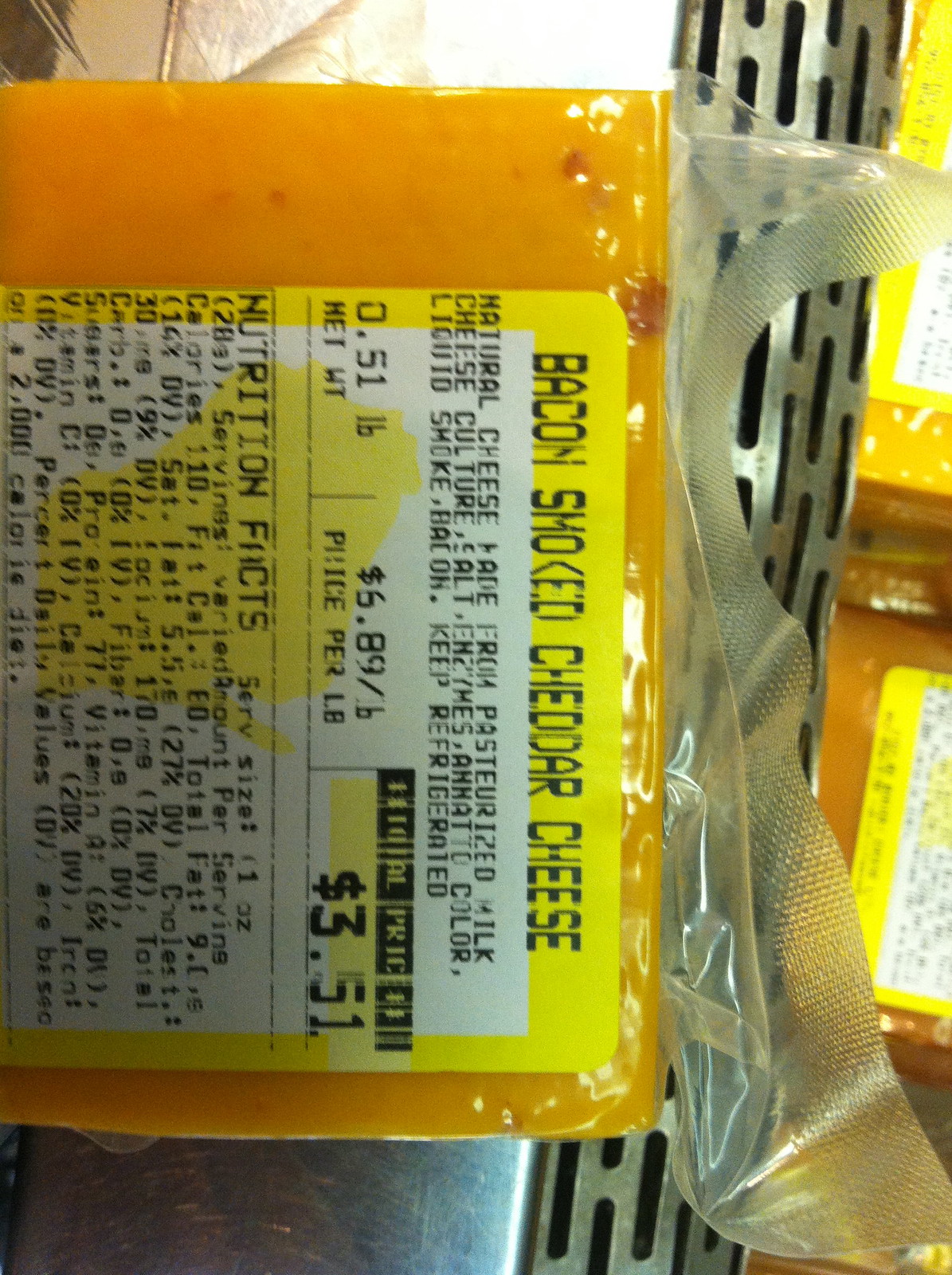A close-up photograph captures the packaging of a bacon smoked cheddar cheese, prominently displayed on a supermarket shelf. The cheese, encased in an airtight vacuum-sealed plastic wrap, showcases its rich orange hue interspersed with visible red bacon bits. The focus of the image is the detailed label, which is designed in yellow and white with black text. This label provides crucial information including a description of the bacon smoked cheddar cheese, a list of ingredients, the cheese’s weight, price per pound, final price, and nutritional data. The photo is taken from a landscape orientation, although the text on the label is slightly angled, making it somewhat challenging to read.